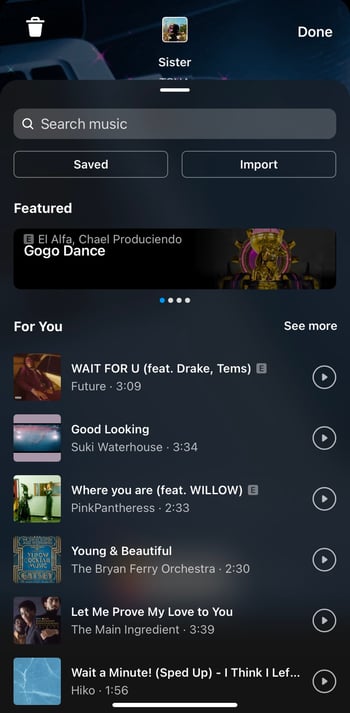A young girl, around 7 years old, dressed in a vibrant pink tutu and white ballet shoes, is standing in the center of a spacious room with large windows allowing sunlight to flood the space. Her sister, a teenager wearing casual clothes, is on the left, holding an acoustic guitar ready to play. Several discarded sheets of paper, likely lyrics or music notes, lie crumpled around their feet, suggesting numerous attempts to perfect a song. Music-related items such as a pair of headphones, a microphone, and some music sheets are scattered across a nearby table. The room has a creative atmosphere, with posters of popular artists like Drake, Willow, and Suki Waterhouse pinned on the walls. Bright and colorful, the scene captures a moment of joyful collaboration and creativity between the siblings.